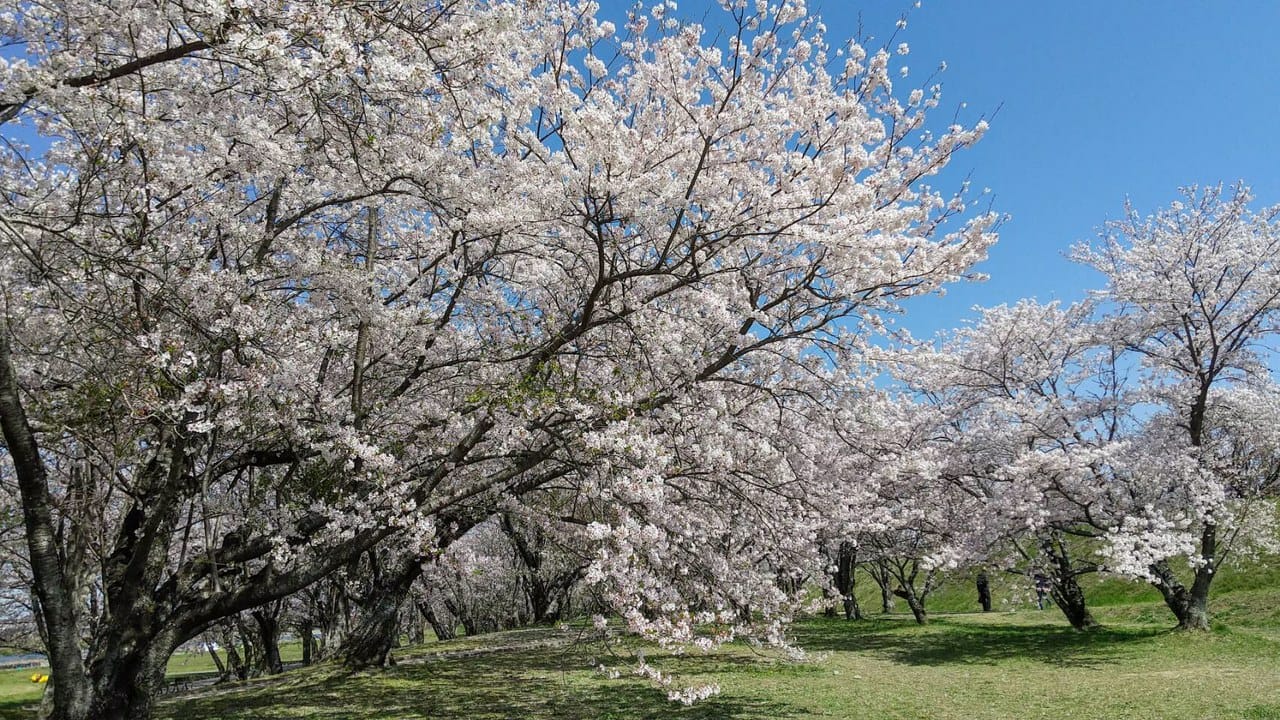In this captivating photo, we see a picturesque outdoor scene featuring a series of low-lying cherry blossom trees with striking white petals, an unusual but beautiful variation from their typical pink hue. These trees are part of what seems to be a park or a grassy field, which gently undulates into a curvy hill. The trees, with their dark bark, are arranged in a row running from left to right, their numerous branches heavily laden with blooms that stand out vividly. The setting is bathed in sunlight, enhancing the brightness of the blossoms and illuminating the fresh green grass below, which is peppered with a few dandelions and possibly some orange flowers in the distant left. A pathway meanders through these trees, adding a charming element to the composition. The sky overhead is a clear, vivid blue, free of clouds and contributing to the serene and cheerful atmosphere. A glimpse of water can be seen in the far left corner, completing this idyllic haven.